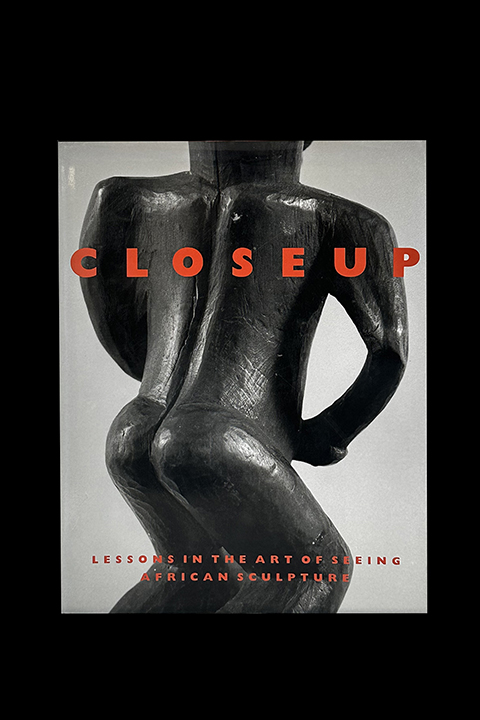The image depicts an old, intricately carved wooden mask, likely of African origin, centered against a completely black background. The mask features a narrow, elongated face with a pointy chin at the bottom and a conspicuous hole at the top of the head, suggesting damage or wear. The mask, predominantly oak-colored with varied shades of dark brown in the carved recesses, gives off an aged appearance. The eyes, devoid of eyeballs, contribute to a sleepy or disengaged expression. The overall style evokes a sense of the mask floating in empty blackness, enhancing its mysterious and solemn aura.